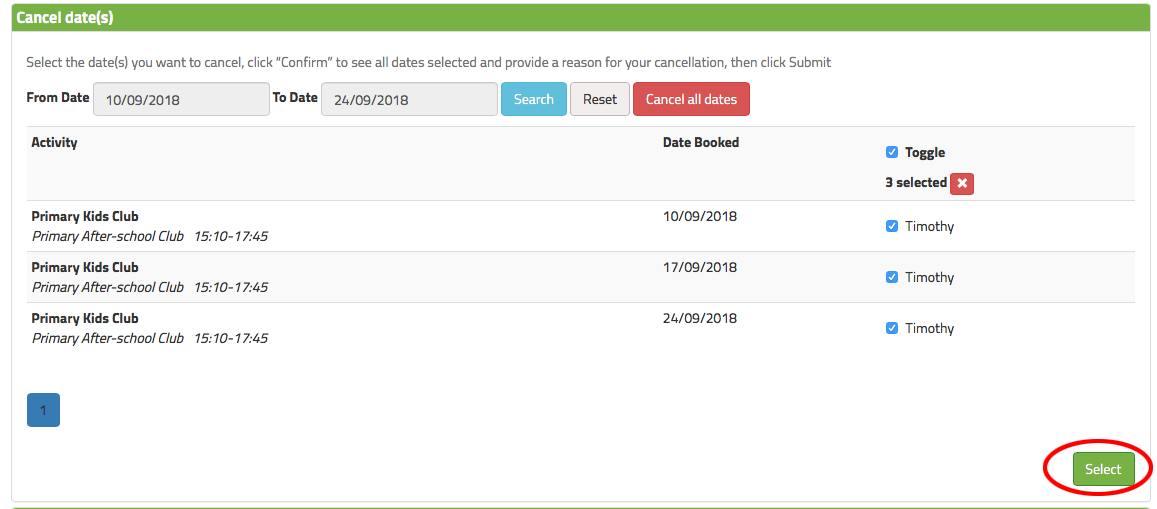The image displays a web interface for canceling scheduled dates for a child's participation in school-related activities. The interface instructs users to select the dates they wish to cancel by ticking checkboxes next to each date and then clicking a "Confirm" button to review the selected dates. Users are also required to provide a reason for their cancellations before clicking "Submit." The interface showcases a list of activities such as the "Primary Kids Club" and "Primary After School Club," with specific dates, September 10, 17, and 24, indicating a weekly frequency. The name "Timothy" is associated with these bookings, suggesting it may be the student's name.

The bottom right of the page features a green "Select" button, highlighted with a manually-drawn circle. Users can search for dates by selecting a "from" and "to" date range and then clicking a blue "Search" button. There is also a "Reset" button and a red "Cancel All Dates" button for additional functionality. The background of the interface is predominantly white with most of the text in black. At the top of the window, there is a horizontal green band providing a splash of color. Overall, the page is designed to facilitate the cancellation of school-related activities, though it is unclear if the cancellations are permanent or temporary.